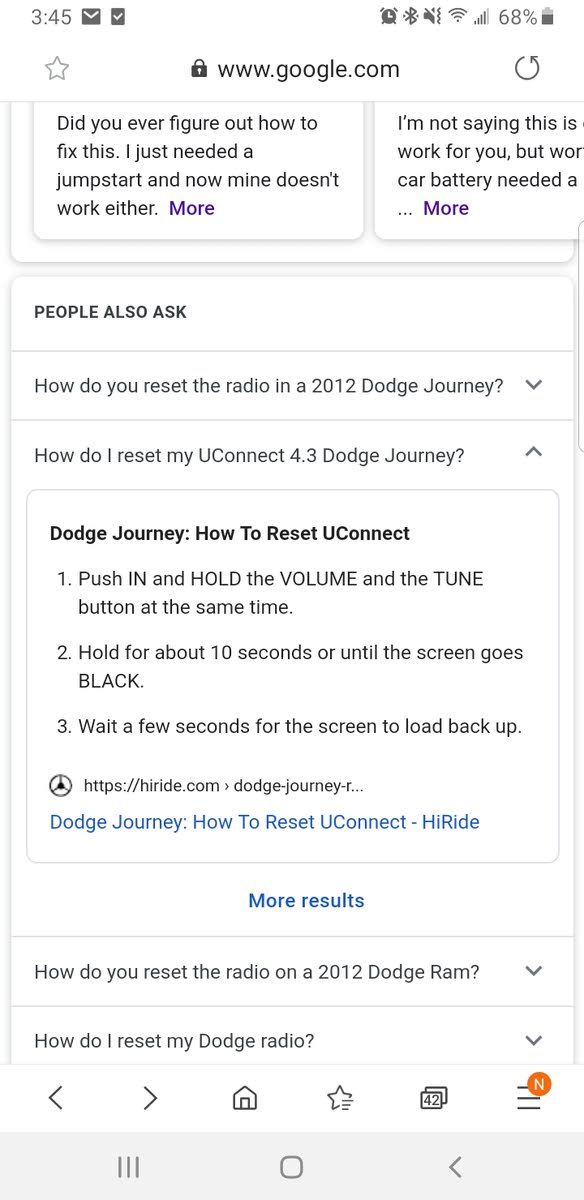A screenshot depicts a Google search regarding how to reset the radio on a 2012 Dodge Journey. At the top of the image, the URL "www.google.com" is visible next to a battery indicator showing 68% and a timestamp reading 3:45. The search query highlighted is, "How do you reset the radio on a 2012 Dodge Journey?". Below, several related questions are listed, such as "How do I reset my Uconnect 4.3 Dodge Journey?", "How do you reset the radio on the 2012 Dodge Ram?", and "How do I reset the Dodge Radio?".

The selected result provides detailed instructions: 

1. "Push in and hold the volume and tune buttons at the same time."
2. "Hold for about 10 seconds or until the screen goes black."
3. "Wait a few seconds for the screen to load back up."

The instructions emphasize specific actions in all caps, indicating their importance. Parts of the options are partially obscured by scrolling and there is an icon resembling a steering wheel adjacent to the instructions. The result source is identified as "HiRide.com," displayed in blue, suggesting a link to further information on the HiRide website.